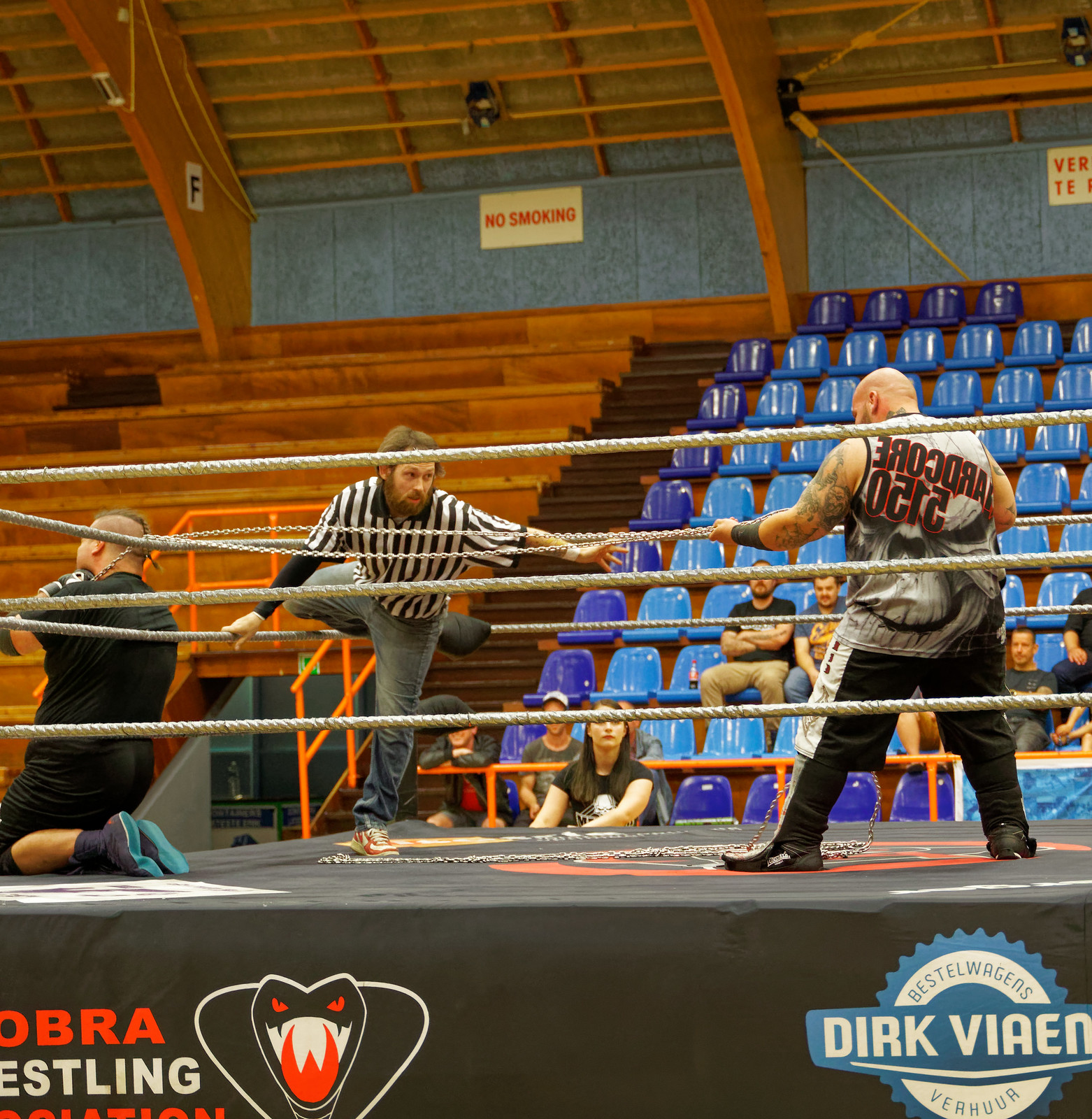In this detailed image from a wrestling match, the scene unfolds in what appears to be a small gymnasium-type auditorium. The main focus is the wrestling ring emblazoned with "Cobra Wrestling" and an image of a cobra snake on the side. The ring itself hosts a dramatic moment: a large, portly wrestler in his 30s, bald and donning a tank top with a skull design, shorts, and high boots, stands ready. Another wrestler is incapacitated, down on his knees by the ropes to the left.

A referee, clad in a traditional striped shirt and jeans with Nike sneakers, is caught in motion, one leg up as he crawls over the ropes into the ring, aiming to reach the standing wrestler.

Surrounding this intense scene, spectators observe from blue plastic seats and brown bleachers. High above, various signs are visible, including "No Smoking" and "Section F." An orange railing marks the boundary area, and another partially obscured sign is seen to the right side. Additionally, there's an advertisement for "Bestel Wagons Dirk Vian," contributing to the local flavor of this enthralling wrestling event.